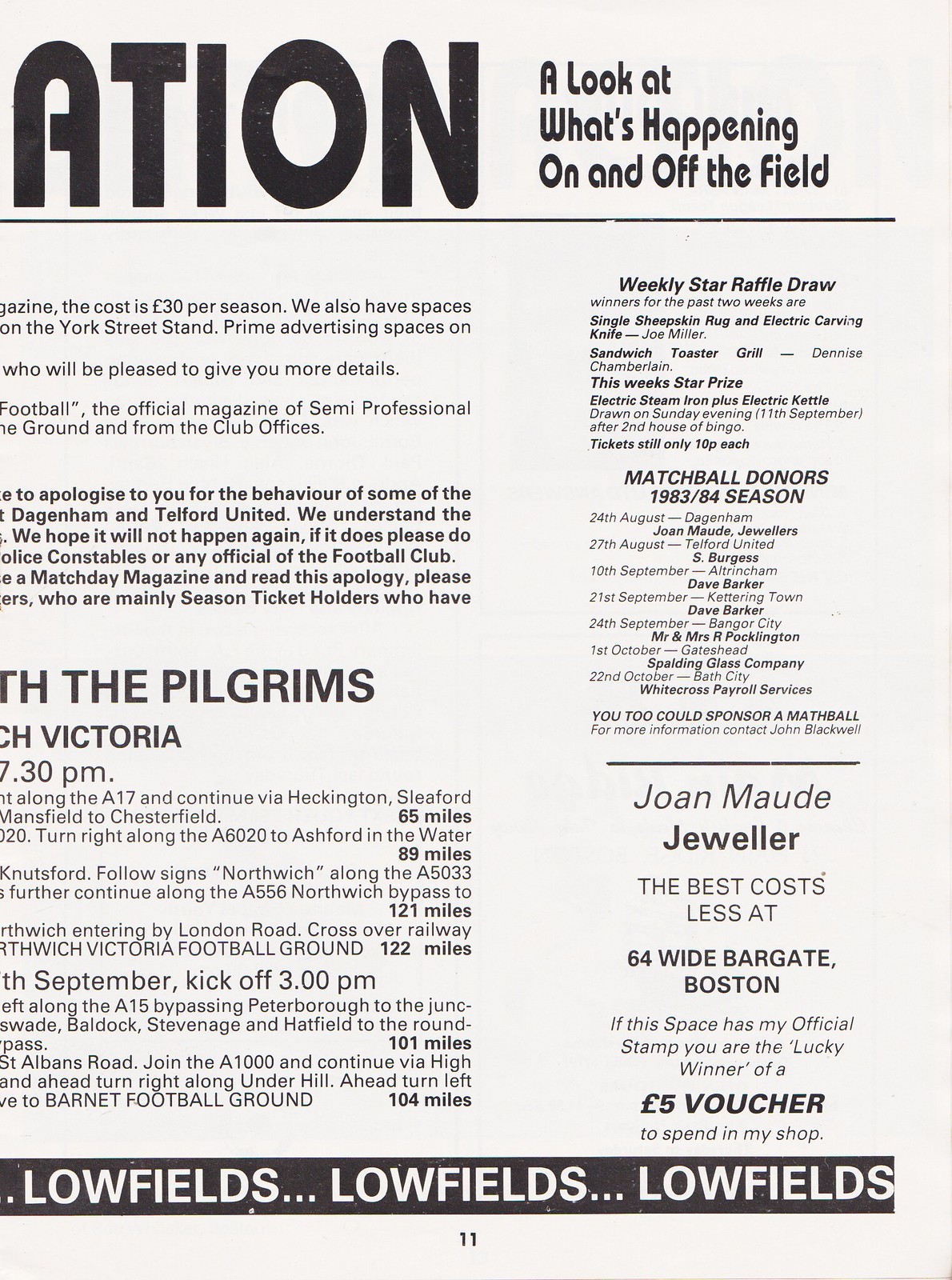The image appears to be a cut-off section of a black and white magazine or program dedicated to a sporting event. The top header, partially visible, reads "ATION," and below it, "a look at what's happening on and off the field." The left side of the page is missing, but the right side provides clear information. It includes details of a "Weekly Star Raffle Draw" with winners Joe Miller and Denise Chamberlain at a ticket price of 10 pence. Mentioned are the matchball donors for the 1983-84 season. Additionally, there is an advertisement for Joan Maud Jeweler, proclaiming "the best costs less at 64 Wide Bargate, Boston." If the advert features an official stamp, it indicates a £5 voucher for the shop. The bottom portion displays a black and white ticker-like banner repeating "Lowfields" in all caps, along with the page number 11. The visible sections include descriptions of prime advertising spaces and semi-professional football details, as well as driving directions for upcoming games, though much of this text is incomplete due to the cut-off.